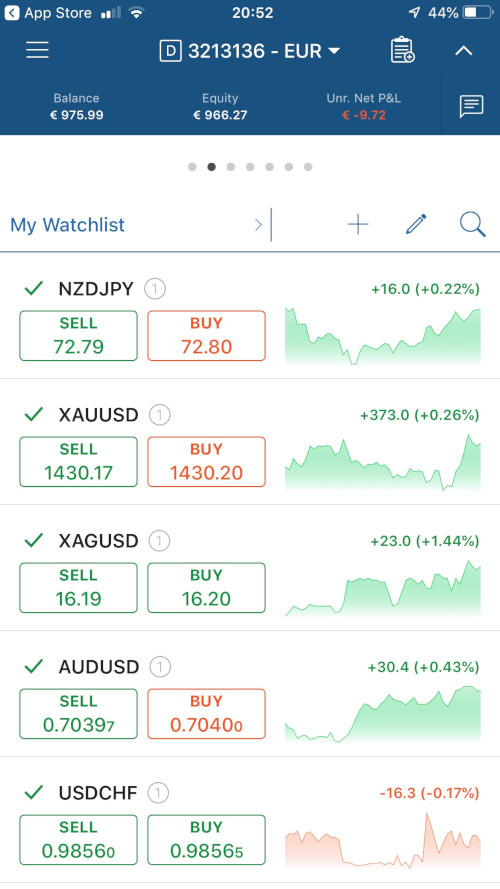**Caption:**

This is a detailed screenshot of a mobile trading app's watch list, primarily focused on currency trading. At the top, within a blue field, there is text indicating "App Store," followed by the time "20:52," a battery percentage of "44%," and a hamburger menu. Below this, we see the user profile "DNS square" alongside the identifier "3213136-EUR," indicating trading is conducted in Euros. A clipboard icon with an up arrow is also present.

Key financial metrics displayed include:
- **Balance:** €975.99
- **Equity:** €966.27
- **Net P&L:** -€9.72 (in red, indicating a loss).

Below these metrics is the watch list section with icons for editing, adding, and searching entries. Various currency pairs are listed, each accompanied by green check marks. The pairs mentioned include NZD/JPY. Each listing has associated sell and buy buttons, displayed respectively in green and red, and a corresponding graph that uses green shading for gains and red shading for losses.

Here are some specific sell and buy prices along with performance data for selected currency pairs:
- **XAU/USD:** Sell at $72.79, Buy at $72.80
- **XAG/USD:** Sell at $16.90, Buy at $16.20
- **AUD/USD:** Sell at $0.70397, Buy at $0.70400
- **USD/CHF:** Sell at $0.98560, Buy at $0.98565

The results for these trades are as follows:
- Gain of +16.22%
- Gain of +3.73%
- Gain of +0.26%
- Gain of +1.44%
- Gain of +0.43%
- Loss of -0.17%

Graphical representations beside each currency pair show green lines and shading for profitable trades, and red shading for losses, offering visual cues at a glance.